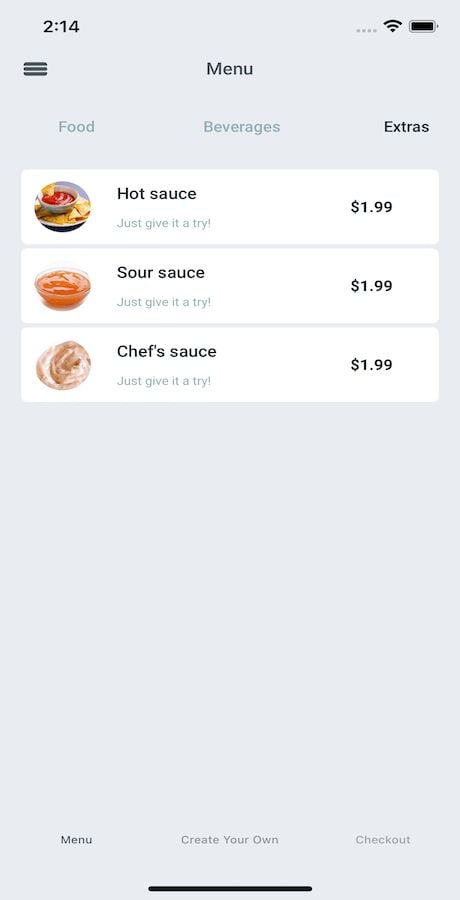This screenshot of a smartphone displays a detailed menu interface of a food-related application. The image shows the time at 2:14 PM in black font located in the upper left-hand corner of the screen. On the upper right-hand corner, there are icons for wireless signal and battery life, both depicted in black.

Centered below the status icons is a menu section, flanked on the far left by a button with three parallel lines, indicating a menu option. This is followed by three horizontally arranged category tabs labeled "Food," "Beverages," and "Extras." The "Extras" category is highlighted in black, indicating the current selection, while "Food" and "Beverages" are displayed in grey font.

Under the category tabs are three detailed product tiles:

1. **Hot Sauce**: Accompanied by a small photograph of the hot sauce on the left, the description reads, "Just give it a try," in grey font. The price is listed at $1.99 on the right.
   
2. **Sour Sauce**: Similar to the hot sauce tile, it features a photograph on the left, with the text, "Just give it a try," in grey font below the title. The price is also $1.99 on the right.
   
3. **Chef Sauce**: This tile replicates the format, including a photograph on the left, and the phrase, "Just give it a try," in grey font. The price listed is $1.99 on the right.

The section displaying these sauce options covers almost halfway down the screen. The lower half features a grey background. At the bottom of the screen, three navigational options are displayed: "Menu" on the lower left, "Create Your Own" in the center, and "Checkout" on the lower right.